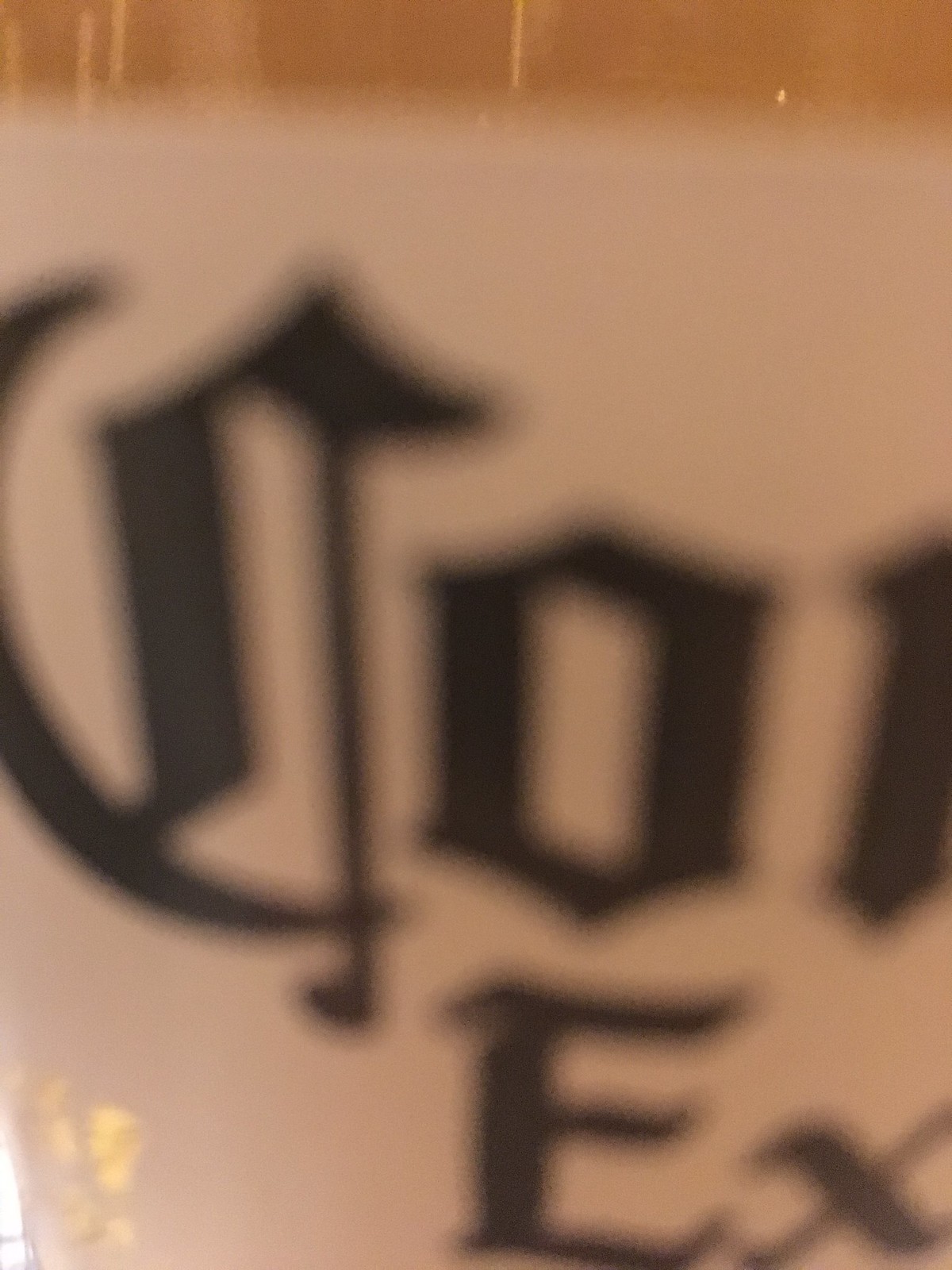A highly magnified, slightly blurred image showcases a classic glass bottle of Corona beer. The close-up perspective reveals only partial elements of the bottle's iconic label: an intricate old English "C" and "O" are distinctly visible, with a hint of the "R" subtly peeking through. Below these letters, an "E" and an "X" can be discerned. The familiar white label and the pale yellow hue at the bottle's neck, indicative of the beer inside, are noticeable, despite the zoomed-in, soft-focus nature of the picture. This intimate portrayal evokes the beer's ubiquitous presence and cultural significance, especially for those who have grown up around this beloved beverage.